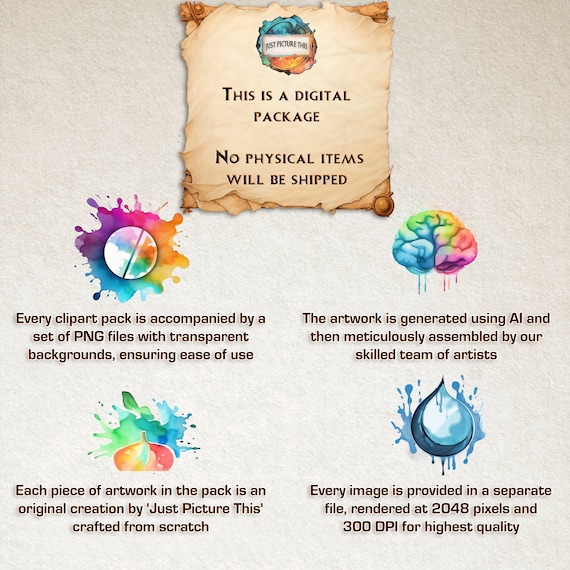The image is an advertisement for a digital downloadable package, set against a gray, textured background resembling an off-white, textured interior wall. Dominating the top of the image is a digital art recreation of an old weathered parchment with browned, rough edges. The parchment, reminiscent of an aged treasure map, features a logo with blue and orange segments and black text stating, "This is a digital package, no physical items will be shipped."

Below this, the image is divided into four quadrants, each containing a blurb that details what the package includes. The top left quadrant showcases a splat graphic, while the top right features a multicolored brain with dripping artwork, indicating that the images are generated using AI and meticulously assembled by skilled artists. The bottom left quadrant displays another splat graphic, elaborating that each piece of artwork is an original creation, crafted from scratch. The bottom right quadrant presents a blue water droplet and assures that every image is provided in a separate file at 2048 pixels and 300 DPI for the highest quality.